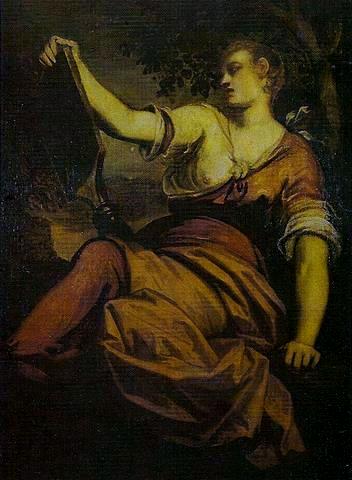The painting depicts a dramatic and almost Baroque-style image of a Caucasian woman lounging back against a tree in a dark, outdoor setting. She has short, light brown, slightly curled hair and a soft, yet contoured facial expression. Her attire consists of a crinkled, orange-rusty red dress, which has slipped off one shoulder, exposing her right breast. The woman's right arm is extended, holding a rectangular object, possibly a mirror, which she gazes into. The tree behind her is silhouetted in dark black with a sparse display of green leaves overhead. The background features a brownish sky, contributing to the overall somber and aged mood of the painting. The dimensions of the image suggest it is a small, rectangular artwork, about two inches wide and three inches tall, with a rich palette of brown, golden, and copper hues that illuminate her yellowish-soft skin tone against the darker backdrop.